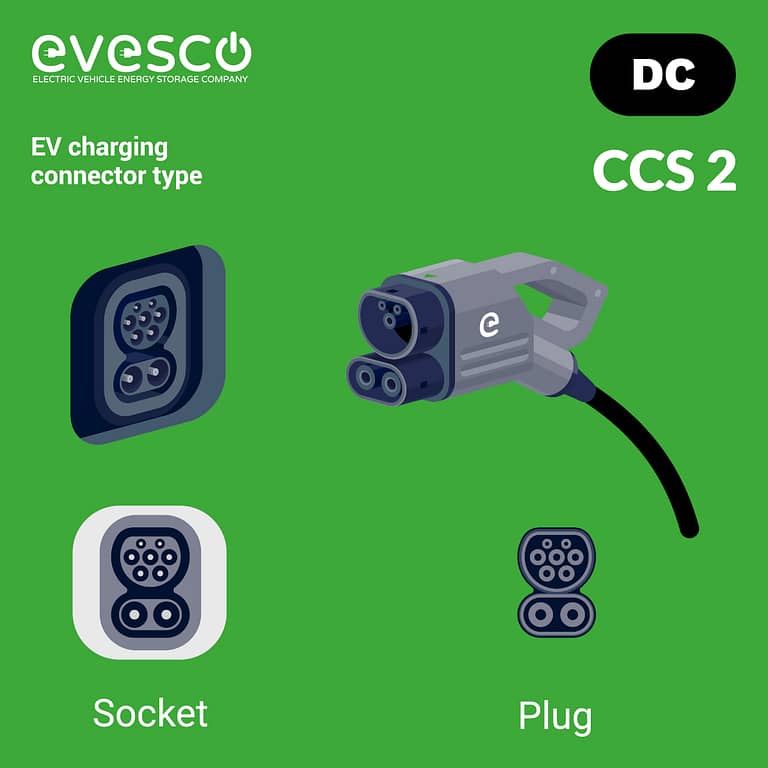The image features a detailed, multi-color print piece associated with Evesco, the Electric Vehicle Energy Storage Company. The layout is vertically rectangular with no border, set against a green background. Detailed white text is displayed in the upper left corner stating "Evesco, the Electric Vehicle Energy Storage Company," with an additional line below reading "EV charging connector type." 

In the upper right corner, a black oval prominently features white text with "DC" and "CCS2" below it. The image includes a detailed infographic displaying various plug and socket types. On the lower left corner, a labeled face diagram of the socket is depicted, while the equivalent face diagram of the plug is shown in the lower right corner. 

The centerpiece of the illustration is a grayish electric vehicle charging device that includes a plug with a distinct handle and a connected black cord. The plug's face has three smaller holes and an intricate detailing of six holes, indicative of the connector's design. Below the plug, a pill-shaped area with two large plug holes is emphasized, which matches the respective design of the socket. This informative piece serves as an educational tool on the different EV charging connector types, illustrating compatibility between plugs and sockets to ensure proper connection for electric vehicle charging.